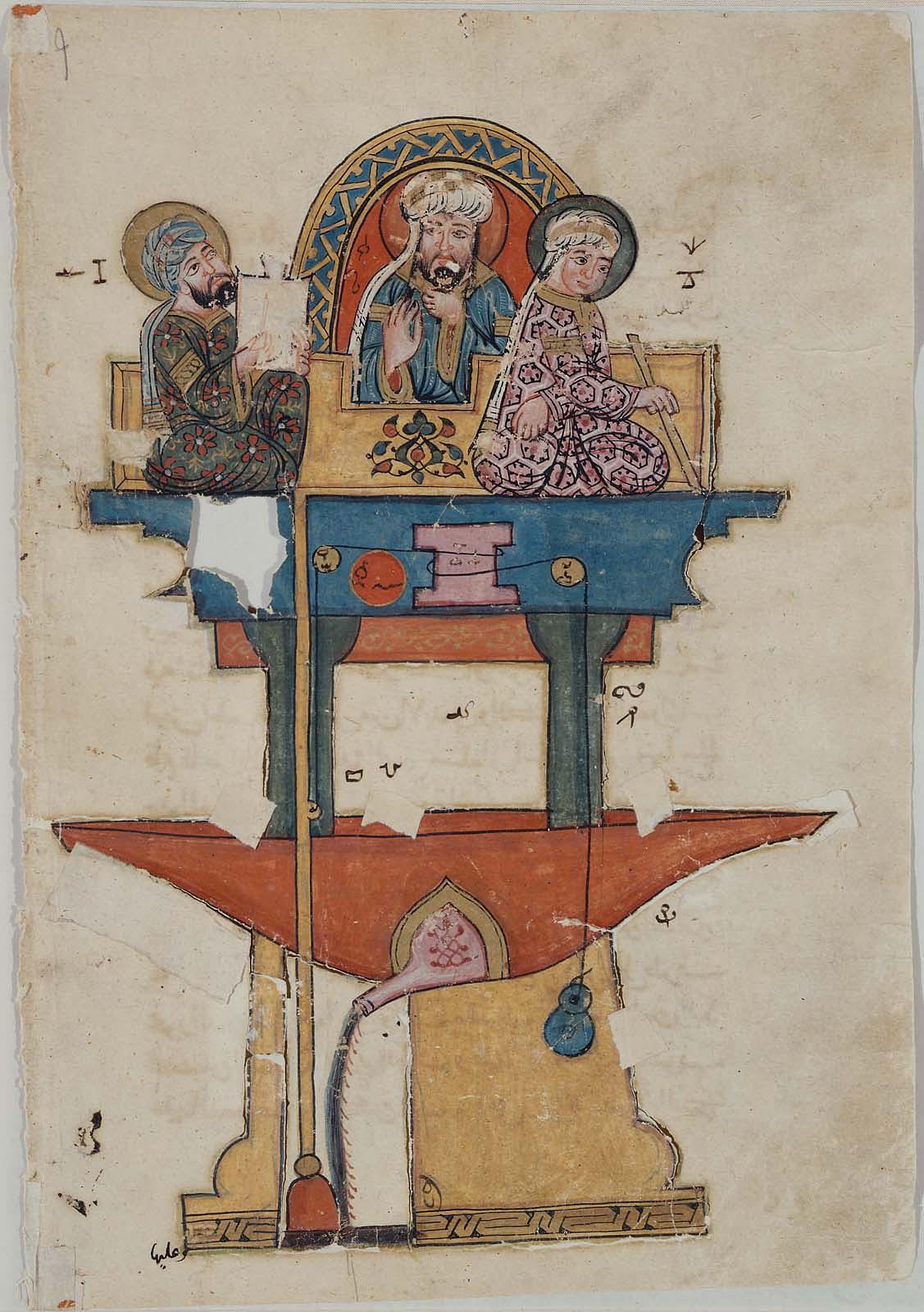The image appears to be a photograph of a Middle Eastern painting, likely on an old parchment. The painting depicts a multi-layered structure or temple with prominent colors such as gold, red, blue, and shades of purple. The artwork features three figures, presumably from a religious context, seated on two landings. The first landing is red, and the second is blue. The central figure, possibly an imam or prophet, is flanked by two others. On the left, a man in a floral red robe and ornate headwear seems to be reading a book and looking upwards. On the right, a woman in a purplish-white robe, also with head covering, is holding a stick or lever. The figures are sitting on a blue pedestal supported by greenish posts and a rust-colored platform, which sits atop a brownish base. The background of the painting is an off-white parchment color, and the image is mounted or placed on a white surface. Some parts of the painting show signs of wear, suggesting it might be from an old religious text or book.